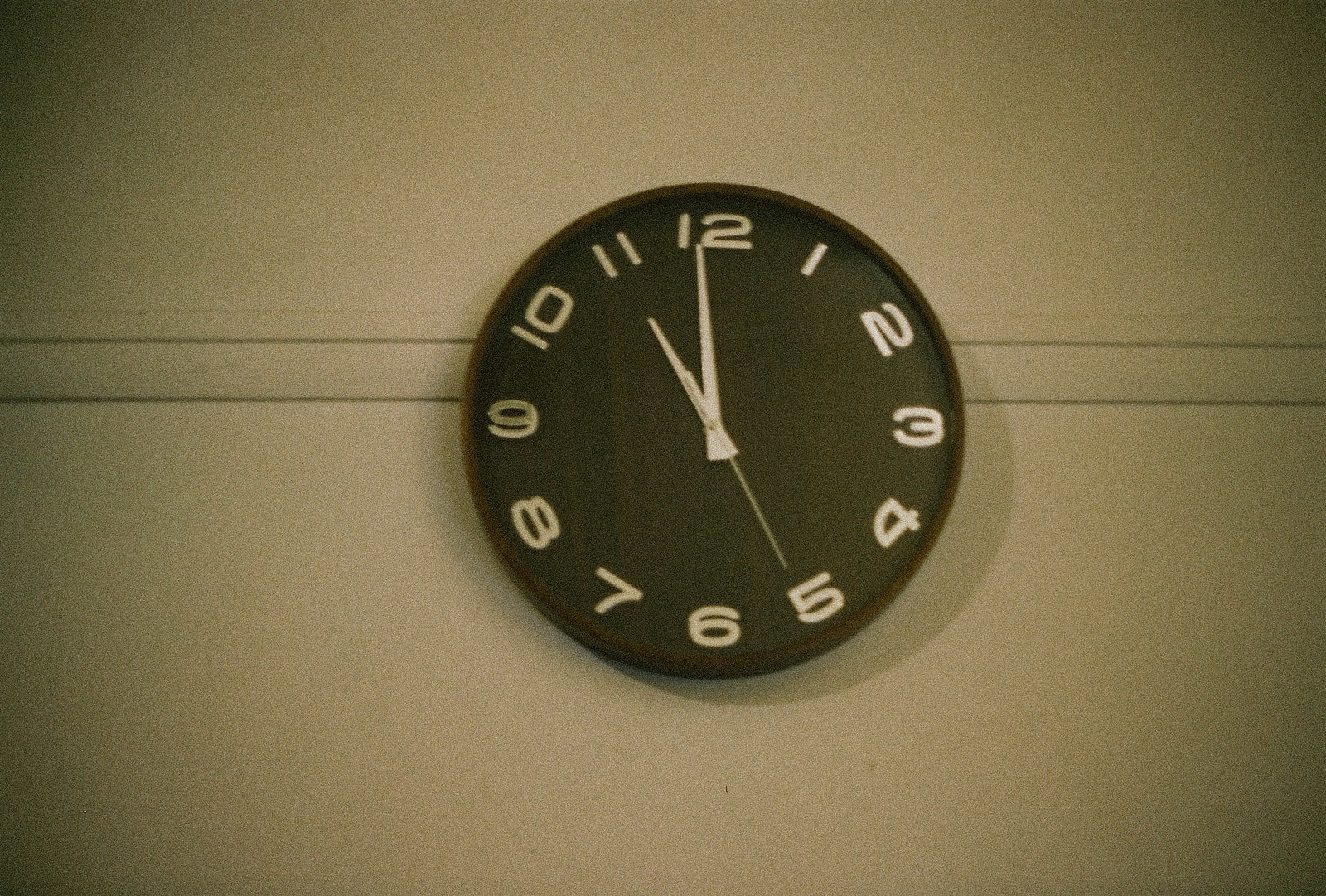The image depicts a wall clock mounted on a beige-tan wall adorned with horizontal molding that has a distinct line running through its center. The wall shows a slight graininess possibly due to the image quality. The clock itself is dark, possibly an army green or a light black, with a black frame and face. It features contemporary white numbers displaying 1 through 12. The hour, minute, and second hands are also white. The clock shows a time of approximately 11:59, with the second hand pointing to the five. The overall appearance of the clock is plain, lightweight, and thin, with a slight shadow at the bottom right hinting at the direction of the light source. The edges of the image have a grayish tint, adding a darker border around the scene.